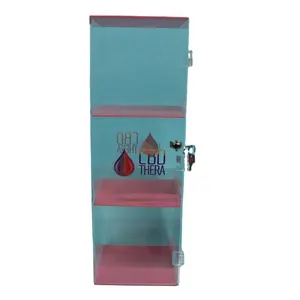The image features a small, clear plastic container, positioned against a white background. The container has a bluish tint with pink shelving inside. It consists of three pink shelves: one on the bottom, one in the middle, and one at the top. The container is slightly wider at the top and narrows down towards the bottom. On the container's front, there’s a label that reads "LBU Thera," accompanied by two droplet graphics; each droplet is half red and half purple, resembling tears or raindrops. Hinges are visible on the right side of the container, suggesting it can be opened, and there appears to be a locking mechanism in the center right. The design hints at a functional, yet visually appealing storage device, possibly for organizing small items like pills or CBD products.